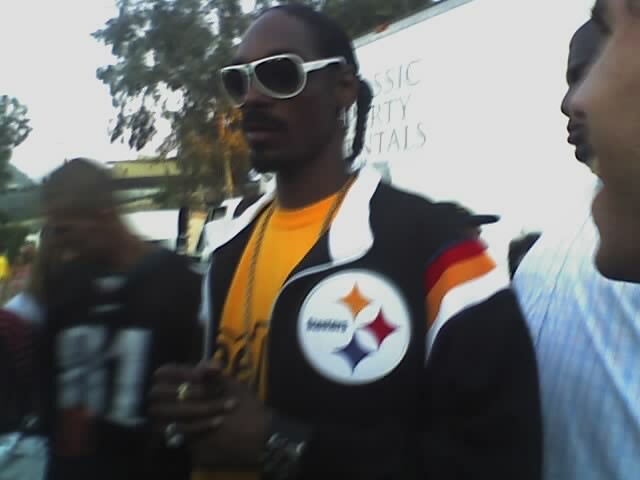This detailed color photograph captures an African-American man standing in the center of the image, adorned with white sunglasses and his hair braided into ponytails and plaits hanging over his ears. He dons an open dark jacket with a distinctive patch on his chest featuring three diamond shapes in yellow, red, and blue, possibly indicating an Olympic or decorative design. His attire also includes a prominent gold chain and thick gold rings on his fingers, suggesting he might be a successful musician. Underneath the jacket, he wears an orange t-shirt with a red, gold, and white stripe on the upper arm. The scene captures him speaking into a cluster of microphones positioned at the bottom left of the frame, while a blurred crowd surrounds him. In the background, there's a banner with "Classy Something Rentals" and a white chalkboard with some illegible writing. The backdrop is set outdoors with green trees and an overcast, cloudy sky. The photograph, either a freeze-frame from a video or a well-timed snapshot, is in landscape orientation and exemplifies a realistic, representational style.